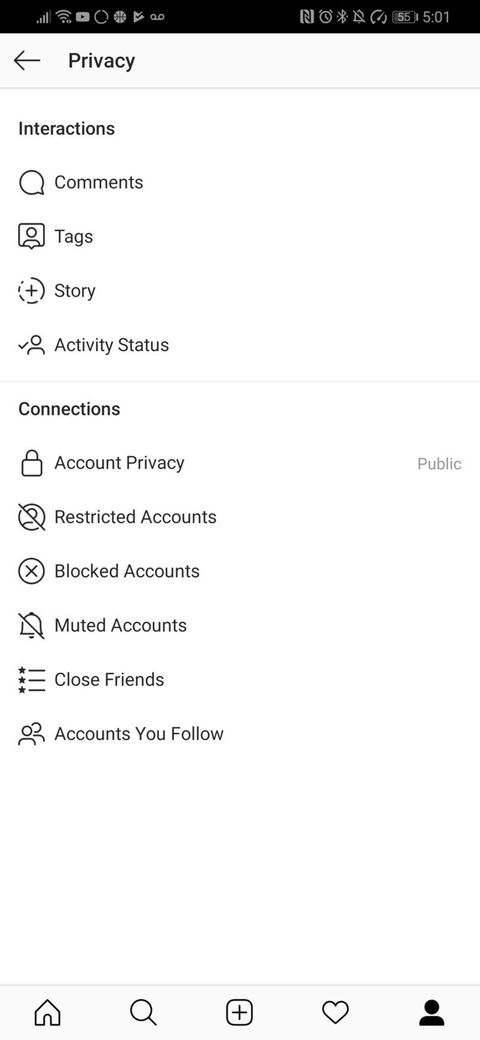This color photograph captures the display of a smartphone held vertically. The phone's screen features the usual indicators at the top, such as signal strength, Wi-Fi connection status, network provider, and the current time. Notably, the device is identified as an iPhone 5S, with an alarm set and Bluetooth enabled. The word "Privacy" is also discernible among the icons.

The main section of the screen has a white background with black text. At the top, an arrow pointing to the left underscores the word "Privacy." Beneath this, the heading "Interactions" is displayed, accompanied by a speech bubble icon labeled "Comments," a bookmark icon titled "Tags," and a circular icon with a plus sign and a partially dotted perimeter marked "Story."

Further down, a silhouette icon with a check mark next to it is labeled "Activity Status." Following this segment, the heading "Connections" appears, under which several options are listed: "Account Privacy," "Restricted Accounts," "Blocked Accounts," "Muted Accounts," "Close Friends," and "Accounts You Follow." The entirety of the content on this screen is indicated to be public.